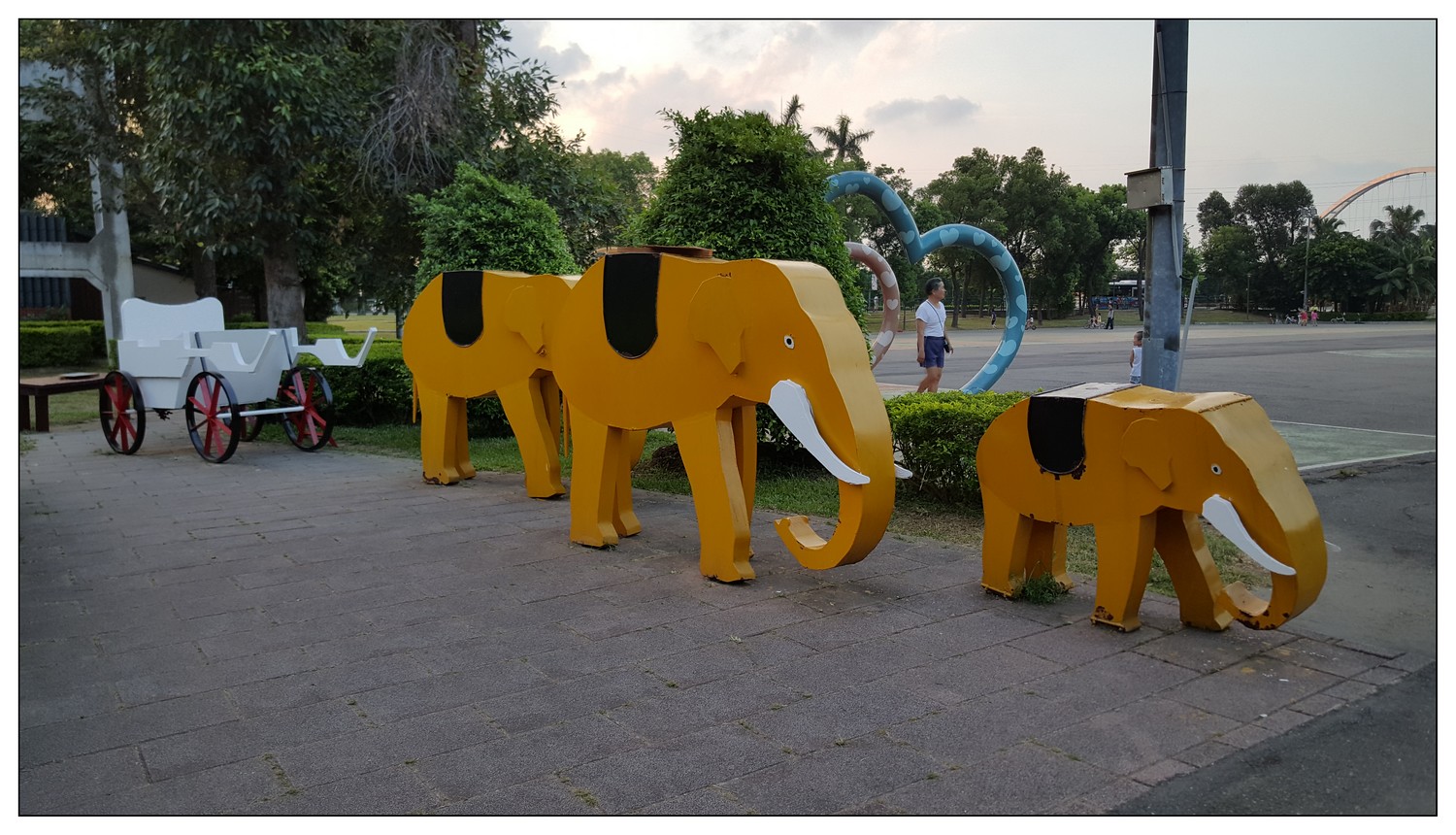The photograph depicts an outdoor scene with a dusk-lit sky in the background, partially visible on the right side with minimal clouds. Beneath the skyline, a row of various trees, including a few palm trees, frames the scene. In the foreground, a large paved area made up of square, reddish-gray bricks extends across the image. Prominently featured on this paved surface are three yellowish-orange elephant statues, each adorned with a black saddle-like stripe across their backs, white tusks, and white eyes. The elephants vary in size, suggesting a familial grouping with one large, one medium, and one small statue. To the upper left of the elephants, there is an old-fashioned white carriage with four black wheels featuring red spokes. A blue heart shape is partially visible among the bushes behind the elephants. Additionally, a Caucasian man wearing a white shirt and blue shorts, possibly with a camera around his neck, is present in the middle of the scene, adding a human element to the composition. The detailed setting suggests the photograph might have been taken at a zoo or amusement park in a location such as Florida.